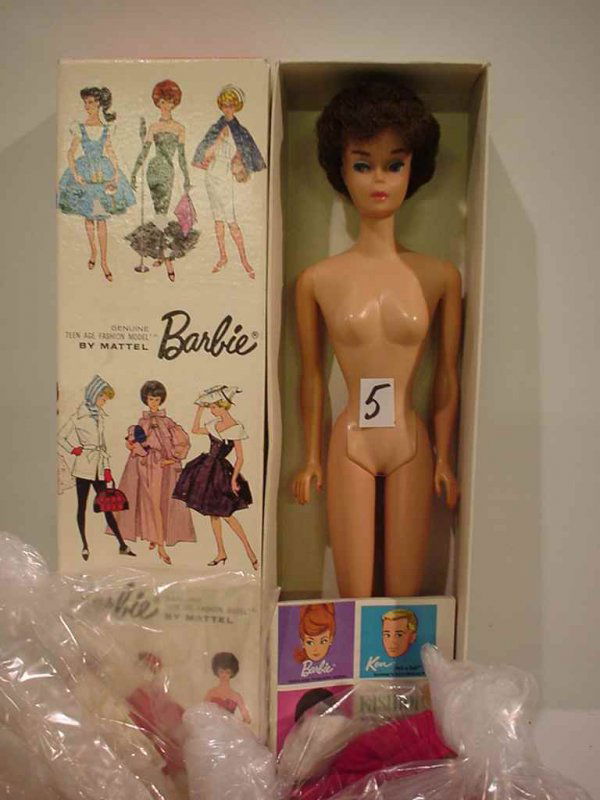This image showcases a vintage Barbie doll, encased in an open cardboard box that sits on a white table. The open lid on the left side features the black-scripted word "Barbie" alongside the Mattel logo, and a series of illustrations depicting different Barbie dolls in various outfits. These outfits range from a Bavarian style dress, a singer or actress ensemble, a midwife uniform, casual clothes, a nightgown, to a traditional dress. The showcased Barbie doll has short brown hair, brown eyebrows, eye shadow, and lipstick. She is unclothed with her arms resting by her sides and has a small white sticker with the black number 5 affixed to her abdomen. Near the bottom of the box, beneath her feet, is a piece of cardboard displaying more Barbie and Ken faces. The box also includes some plastic wrapping, the contents of which are not specified.